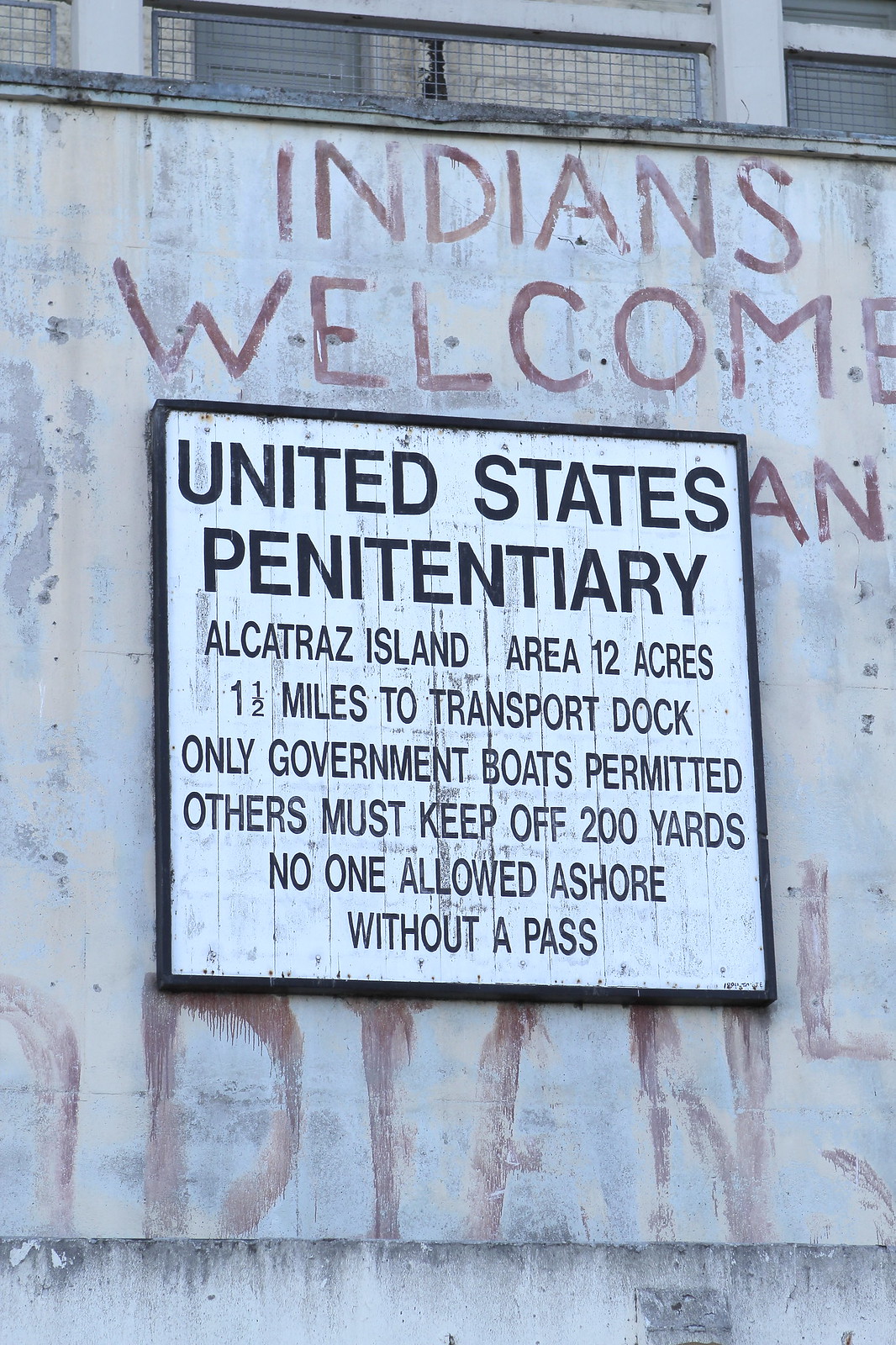The image showcases a worn-out gray concrete wall with visible cracks, featuring a prominent white plaque bordered in black block letters. The plaque reads: "United States Penitentiary, Alcatraz Island, area 12 acres, one and a half miles to transport dock, only government boats permitted, others must keep off 200 yards, no one allowed ashore without a pass." Above this plaque, spray-painted in uppercase letters, are the words "Indians Welcome" in a reddish-brown hue. The weathered background includes partially visible windows and hints of additional indistinct spray-painted text below the plaque.